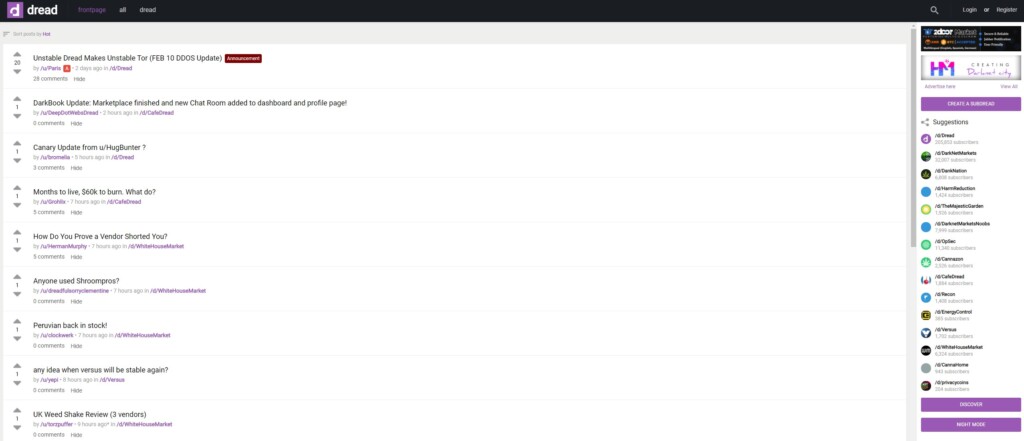This image is a screenshot of a user interface that appears to be from a website or app named "Dredd," identifiable by its distinctive logo featuring a lowercase 'd' with a notch in the lower left part and a purple square next to it. The screen shows a black header bar adorned with several indistinct options, a login button, and a search bar on the right side. Below the header is a list of options marked by up and down arrows on the left side, possibly indicating forum topics or feedback suggestions. Some visible options include "Unstable Dredd makes unstable something," "Dark book update," "Marketplace finished," "New chat room added," and "Canary update." There are approximately eight items in this list, but the text is challenging to read due to its small size and the numerous white space areas. The interface suggests a feedback section where users can upvote or downvote topics, provide complaints, or offer recommendations to developers. On the right side of the screen, there appears to be a menu option, potentially displaying currently logged-in users. Overall, the layout seems to depict a forum-like environment dedicated to user feedback and interaction with developers.